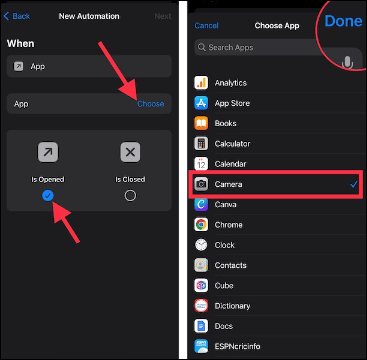The image consists of two juxtaposed smartphone screenshots detailing the setup of an automation task. 

In the left screenshot, the user is in the process of creating a new automation. The screen's header reads "New Automation," and a red arrow directs attention to the "Choose" button associated with the "App" option. The text at the top left corner, "When App," indicates that this automation step is contingent upon an app's activity. At the bottom, another red arrow points to the "Is Opened" option, which is marked with a lit blue check mark, signifying selection. This implies that the automation will be triggered when a specific app is opened.

In the right screenshot, the user has pressed the "Choose" button, bringing up a list of all installed apps on the device. The "Camera" app is highlighted with a blue check mark and outlined in a red rectangle, indicating its selection. Additionally, a red circle emphasizes the "Done" button at the top right corner of the screen. This visual suggests that the user intends to create an automation that activates whenever the Camera app is opened, although the specific action to follow remains unspecified.